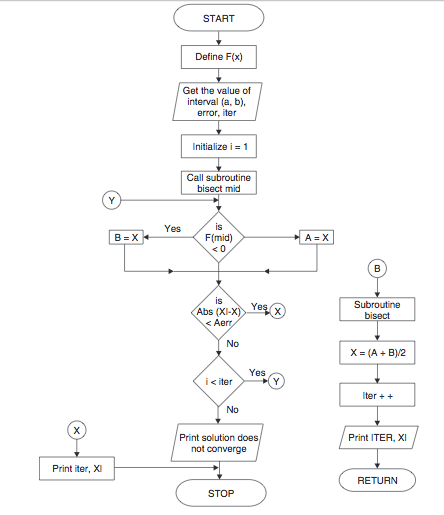The image is a detailed flowchart in portrait layout, featuring black text on a white background with no defined borders. At the top, there's a button labeled "Start," followed by arrows directing downward to sequential steps. The steps include: "Define f(x)," "Get the value of interval [a, b], error," "Initialize i = 1," and "Call subroutine bisect_mid." Below this, there's a decision point marked "Is F_mid," leading to branches labeled "B = X" and "A = X" that reconverge onto steps named "Is abs" and "I < ITER." From here, it proceeds to a step that reads "Print: solution does not converge," concluding with a "Stop" button. To the right of this linear flow, there's a smaller subroutine flowchart starting with "B," then moving through "Subroutine bisect," "X = (A + B) / 2," "ITER++," "Print (ITER, xi)," and ending with "Return."